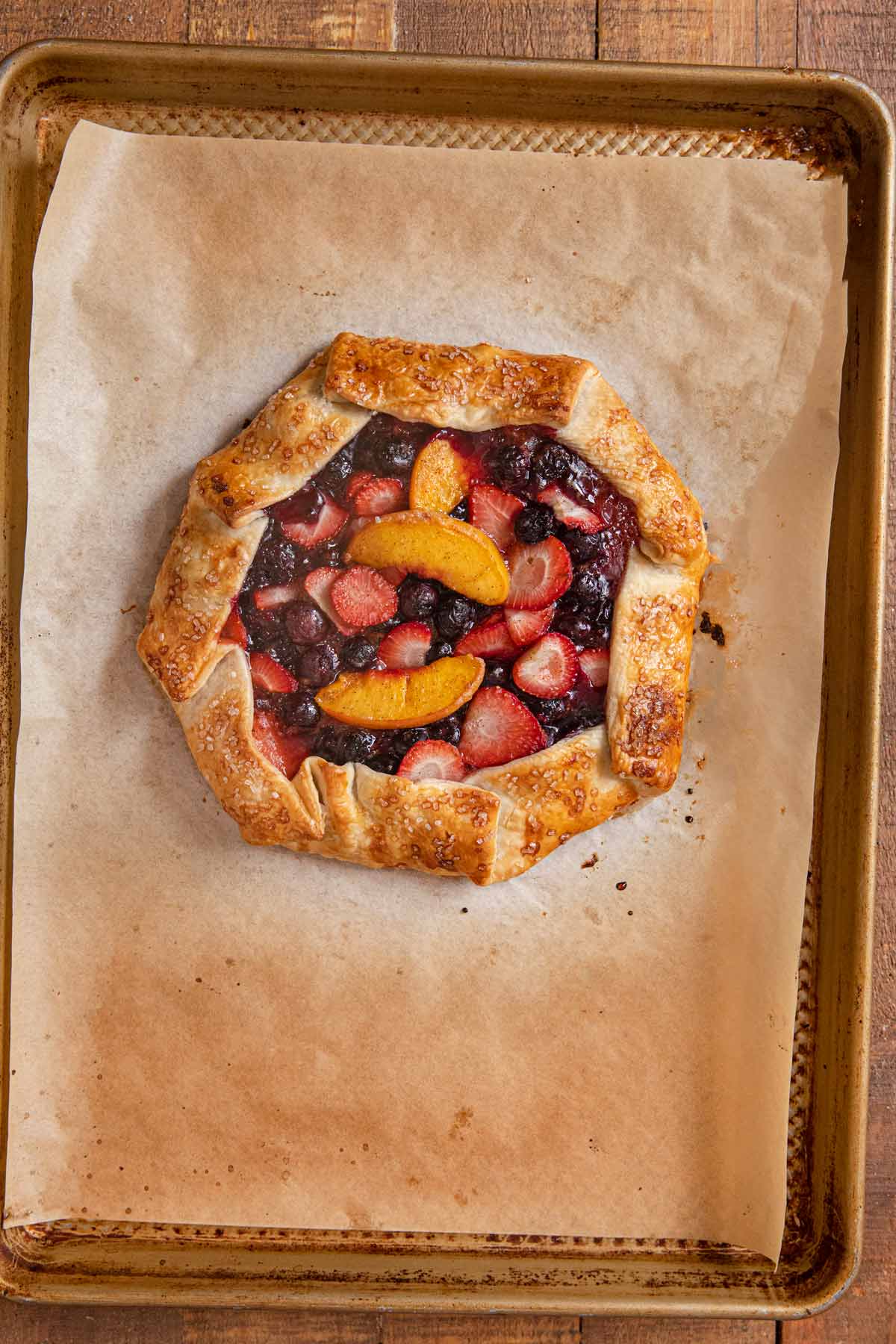Displayed on a rustic wooden table is a freshly baked fruit tart, elegantly presented on a timeworn copper-colored baking sheet covered with tan parchment paper that has browned slightly from the heat. The fruit tart itself is shaped into a unique octagon, with its beautifully browned, crusty edges folded up about an inch, possibly basted with egg to achieve its shiny finish. At the center of the tart, a delightful array of fruits including strawberries, cherries, blueberries, and peaches nestles atop a layer of jam, creating a vibrant and appetizing centerpiece. The crust is sprinkled with sugar, enhancing its visually appealing, golden texture. Overall, this perfectly baked dessert looks irresistibly delicious.